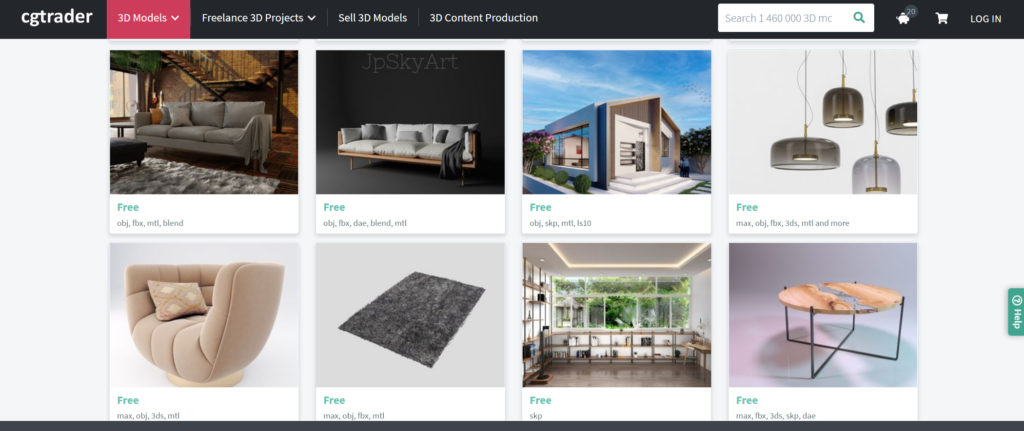The screenshot captures the homepage of the CGTrader website, a platform dedicated to 3D models. The image features a black navigation bar at the top, prominently displaying the CGTrader logo in white. The navigational options include a red-highlighted tab labeled "3D Models," indicating the current selection. Adjacent to this are tabs for "Freelance 3D Projects," "Sell 3D Models," and "3D Content Production." To the right, there is a search bar with a placeholder text stating "Search 1,460,000 3D models," followed by two icons, an unidentifiable one and a shopping cart icon, and a "Login" button.

Below the navigation bar, under the highlighted "3D Models" tab, is a selection of 3D models presented as thumbnails. The first row includes:
1. A loft apartment interior focusing on a couch offered in multiple file types: OBJ, FBX, MTL, and Blender, listed as free.
2. Another couch, also free, by JP Sky Art.
3. An exterior view of a home, which is free as well.
4. Four glass pendant lights hanging, available for free.

The second row features:
1. A soft, cup-like beige chair, free of charge.
2. A gray rug, also free.
3. An extensive free kitchen shelf system.
4. A round table on the far right, available for free as well.

The screenshot is framed by a black bar at the bottom, completing the visual interface of the CGTrader homepage.